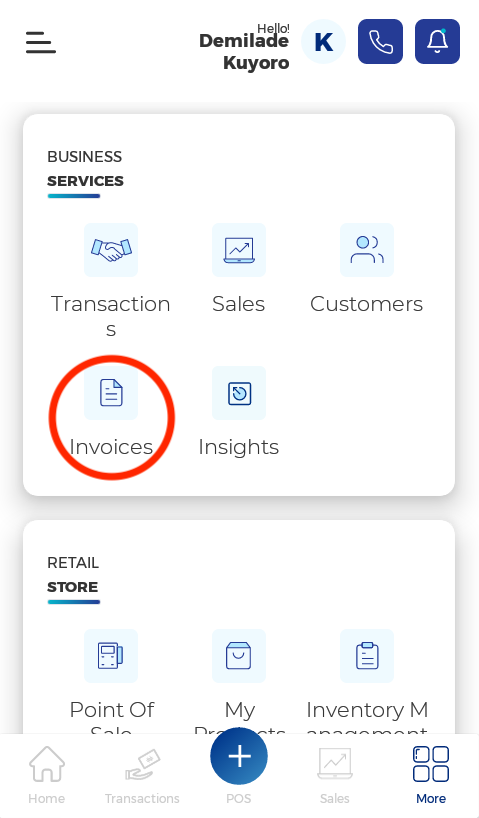The screenshot features an app interface captured on a cell phone. At the top, there are three horizontal lines stacked vertically, serving as the option menu button, and they are colored black. Next to it, on the right, the phrase "Hello, Demilade Kuyoro" is written in black text. Beside this greeting is a small light blue circle with the letter "K" in dark blue at its center.

Adjacent to this, there are two icons: a phone and a bell, the latter representing notifications. These icons are depicted in white against a dark blue background.

The main section of the screenshot has a white background with the heading "Business and Services" in black text. Below this header, there are various service options listed: "Transactions," "Sales," "Customers," "Invoices," and "Insights." Notably, the "Invoices" option is highlighted with a red circle around it.

The lower part of the screenshot is labeled "Retail and Store," offering additional, albeit partially visible, options related to retail services.